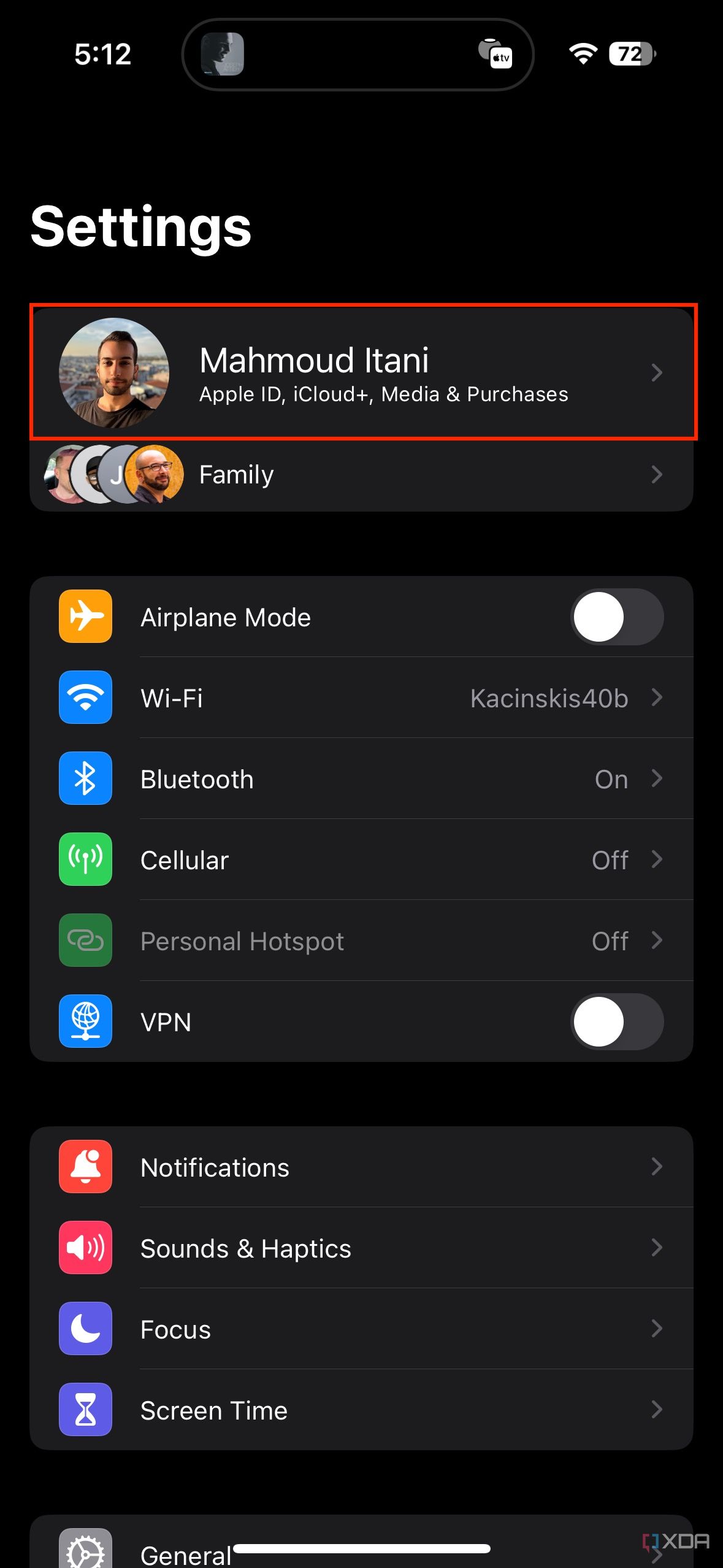This image is a detailed screenshot of the Settings page on an iPhone. 

At the top of the page, the user's profile is displayed, showing the name "Mohamed Atani." Directly beneath the name, there are options related to Apple ID, iCloud, Media & Purchases. Additionally, there is a "Family Sharing" option indicating four other members are connected.

Just below the profile section, various connectivity options are listed:
- Airplane Mode is switched off.
- The device is connected to a Wi-Fi network named "K-A-C-I-N-S-K-I-S 4-0-B."
- Bluetooth is turned on.
- Cellular data is turned off.
- Personal Hotspot is disabled.
- VPN is also turned off.

Further down, additional settings are displayed, including Notifications, Sounds & Haptics, Focus, Screen Time, and General.

The status bar at the top of the screen shows it is 5:12 PM. Icons indicate the battery level is at 72%, and both Wi-Fi and cellular signal strengths are full.